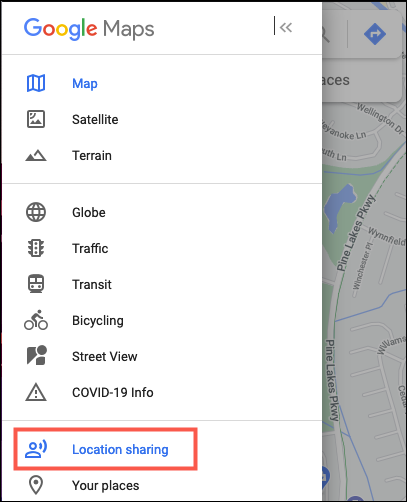This image is a screenshot of the Google Maps mobile interface. Dominating the screen, approximately 80% of it, is a navigation panel that slides out from the left side. This panel is titled "Google Maps" and features various options to enhance user navigation, including arrows at the top. In the background, the faint outlines of a couple of streets are visible, along with part of the familiar Google Maps search bar at the top, complete with a blue button typically used to initiate a search.

Highlighted within the navigation panel is a red square emphasizing the "Location Sharing" option, indicating a focus on or concern for location sharing features. Additionally, "Map" and "Location Sharing" have their text in blue, drawing further attention to these elements. Other selectable features include "Satellite," "Terrain," "Globe," "Traffic," "Transit," "Bicycling," "Street View," "COVID-19 info," "Your places," and more, reflecting the comprehensive nature of Google Maps’ functionalities.

This screenshot appears to be from a regular user’s app rather than a developer's version, suggesting that location sharing is a standard feature aimed at promoting user awareness of their shared locations and its potential implications.